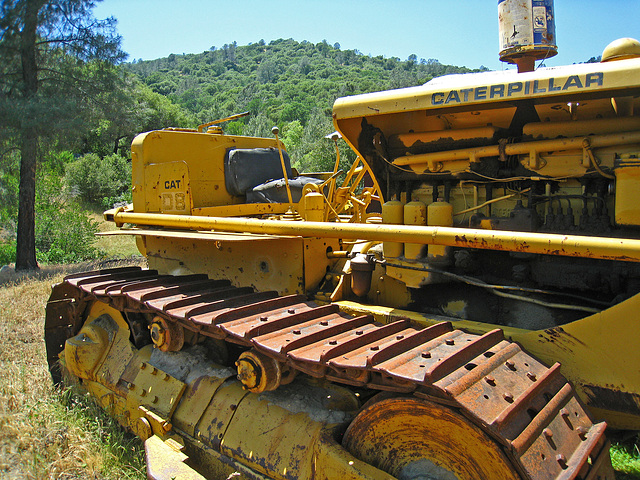This photograph features an old, yellow Caterpillar construction vehicle, likely a backhoe or bulldozer, showing signs of extensive use and weathering. The vehicle, positioned with a side profile stretching to the right side of the image, prominently displays "CAT 08" on both the front and near the seat. Its structure includes large, rusted tank tracks and a worn black seat, indicative of heavy utilization. The bulldozer is nestled in a field with a mix of live green and dead beige grass at the bottom left. Surrounding the field, the scene transitions into a wooded area on the left and the top of the image, with numerous trees and a tree-covered hill in the background. The sky is a clear blue, suggesting a peaceful natural setting. Additionally, the vehicle appears dirty with black grease smears around the treads and rust on various parts, further emphasizing its age and use. On top of the equipment, there's a flipped paint can, adding to the rustic and rugged appearance.